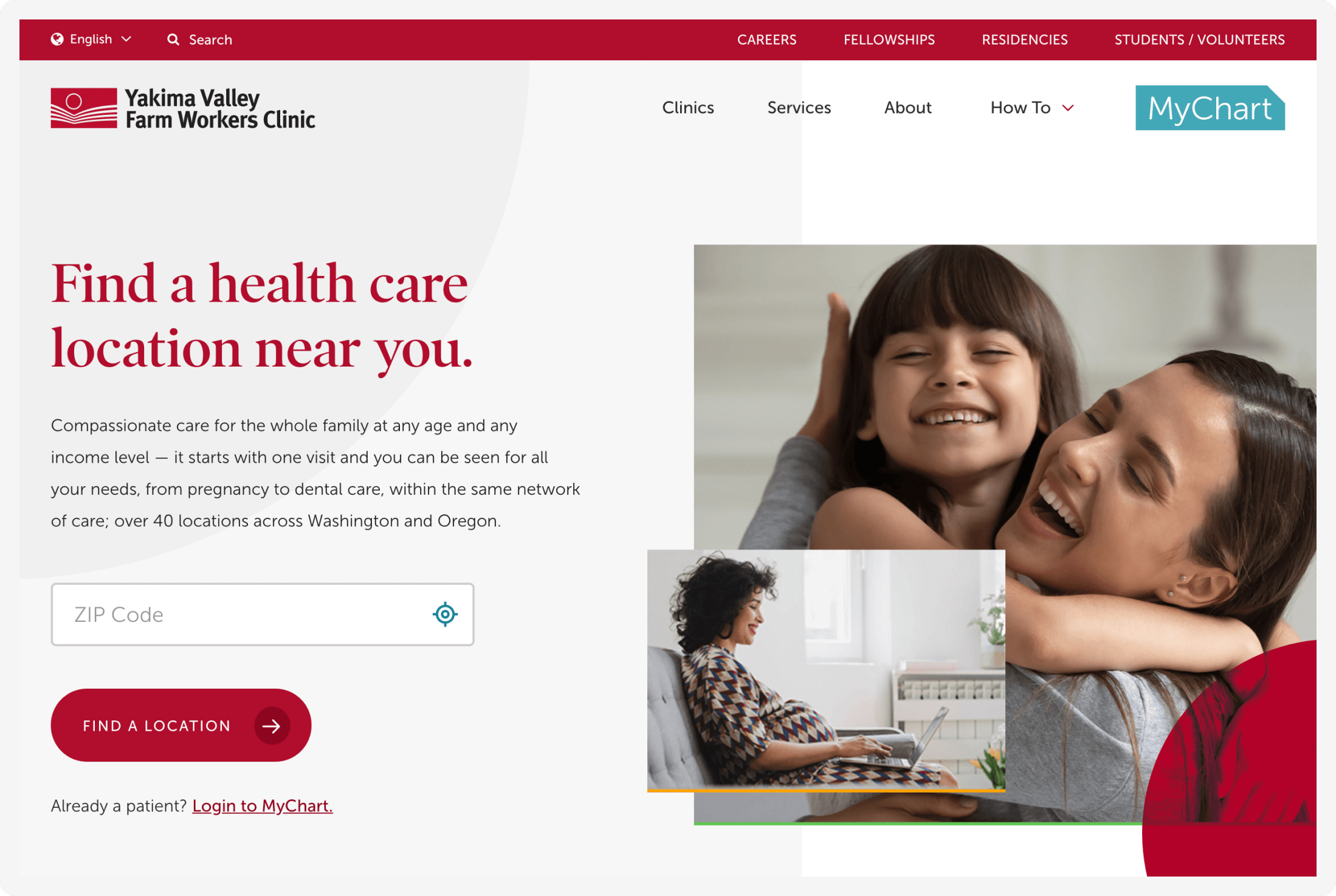The website for the Yakima Valley Farm Workers Clinic is designed to cater specifically to the farm workers of the Yakima Valley area, which has a significant Hispanic population. Dominating the top of the homepage is a full-width red rectangular bar. Within this bar, white text options allow users to select their preferred language, with the default highlighted as English, accommodating multiple ethnicities. Accompanying this is a search bar, identifiable by a small magnifying glass icon and the word "search." Toward the right end of this red bar, there are four drop-down menus titled: "Careers," "Fellowships," "Residences," and "Student Volunteers."

Below this bar is the Yakima Valley Farm Workers Clinic logo, featuring a stylized red sun setting behind red hills, accentuated with white lines. Adjacent to the logo, there are four primary drop-down menus: "Clinics," "Services," "About," and "How To," guiding users to various sections of the site.

This layout and visual design cater specifically to farm workers of the region, providing ease of access to important resources and information.